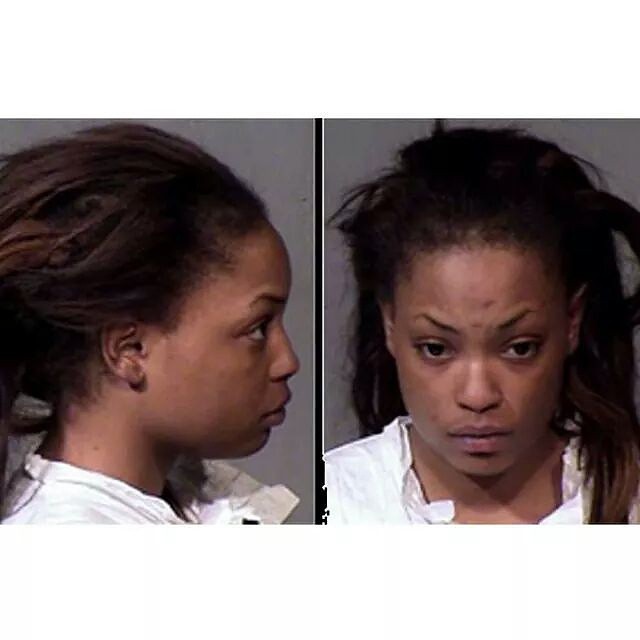This full-color photograph captures two separate mugshots of a young African-American woman, probably in her 20s. Her light brown complexion suggests she is of African-American descent. In both images, she is wearing a plain white shirt. Her long, disheveled black hair, featuring some braids, cascades over her left shoulder and back. The left image showcases her right profile, revealing an open collar and an ear devoid of jewelry. Her expression is somber and bewildered. The front-facing image, placed on the right side, displays her looking slightly downwards. Notable marks, possibly bruises, are visible between her eyebrows, indicative of some form of distress. The neutral gray background further emphasizes the stark reality of the mugshot setting.